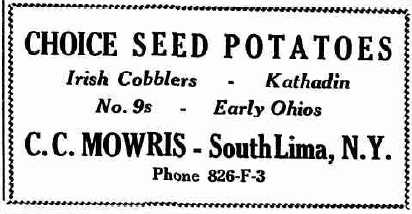The advertisement appears to be a scan of an old-fashioned, text-only ad from a newspaper or magazine, presented with a white background and bordered by a rectangular, wavy line resembling rope. Across the top in bold, uppercase letters, it reads "CHOICE SEED POTATOES." Below this, in smaller italic print, it lists various types of potatoes: "IRISH COBBLERS," "KATHADIN," "NUMBER NINES," and "EARLY OHIOS." At the bottom, in larger capital letters, it reads "C.C. MORRIS," followed by "South Lima, New York" in mixed upper and lower case. The contact phone number is "826-F-3."